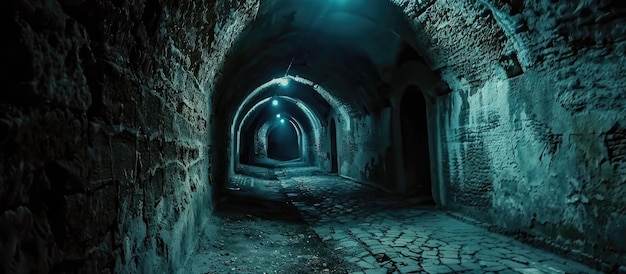The image depicts a long, dark subterranean tunnel with an arched ceiling. The tunnel extends approximately 50 to 100 feet into the blackened distance, illuminated only by small, cold blue electric lights spaced at regular intervals along the center of the ceiling. The walls, made of deteriorating concrete and brick, show signs of cracking and wear, with colors varying from reddish to gray, and streaks of white likely due to lime deposits from age. On the right side of the tunnel, there are several arched doorways leading into other dark passages. The floor varies in texture; parts are dirt-covered with scattered pebbles and broken concrete, while others appear to be made of worn, interlocking cobblestones. The overall atmosphere is mysterious and foreboding, strongly suggesting it is an old, neglected structure.